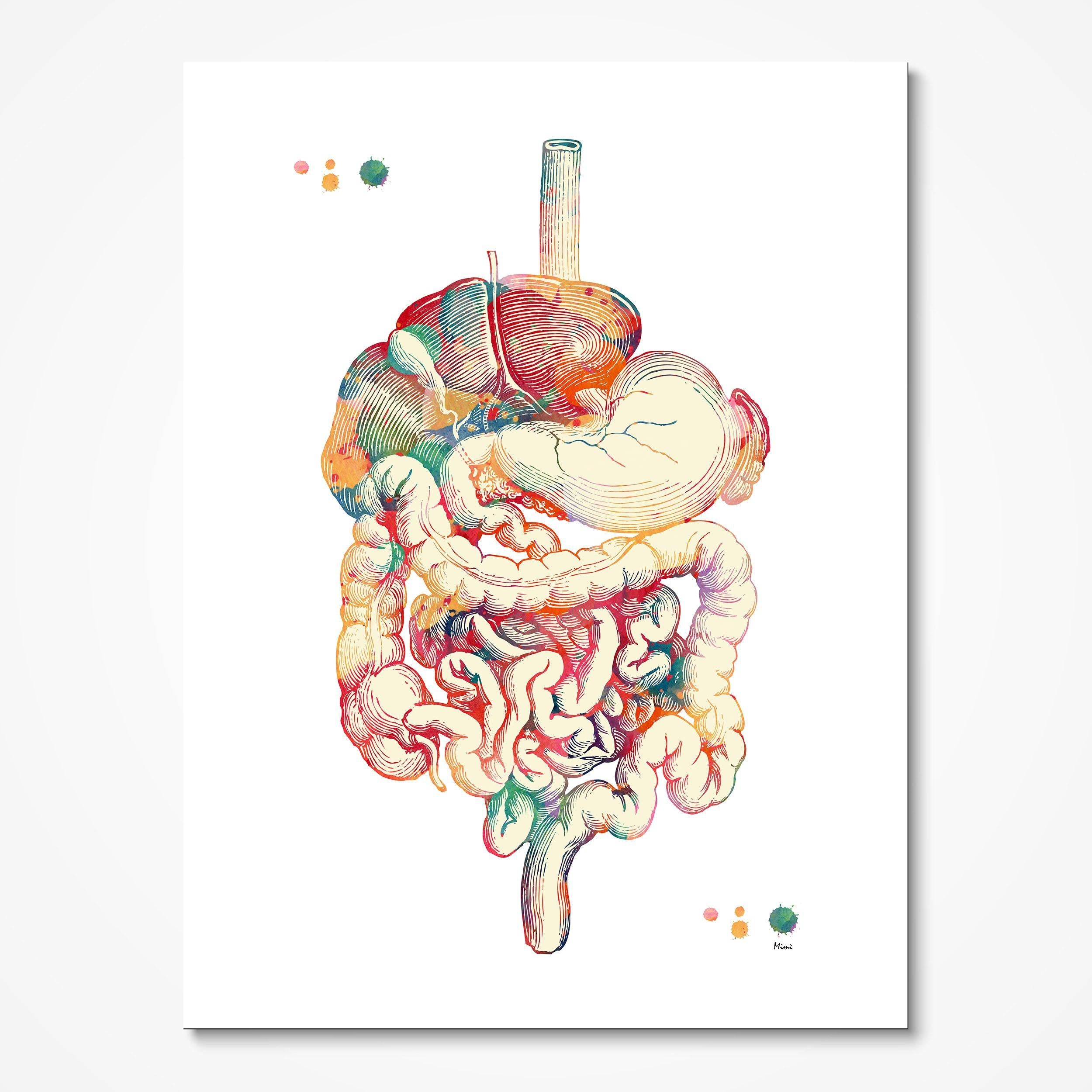The image is an artistic, computer-enhanced illustration of the human digestive system, prominently displayed against an off-white wall. The artwork likely uses pen and ink, enhanced with a vibrant, rainbow palette of reds, greens, blues, and purples. At the top of the image, a green part surrounds a red and orange section, capped by a circular tube. Below this, on the right side, there is a light yellow stomach. The small and large intestines are depicted beneath the stomach, with the larger intestine encircling the smaller one in a looping pattern. The top left and bottom right corners of the image feature additional paint splotches, one green circle surrounded by three orange circles, along with an illegible artist’s signature. This piece could be a mock-up or a print potentially for sale and resembles diagrams typically found in biology textbooks.